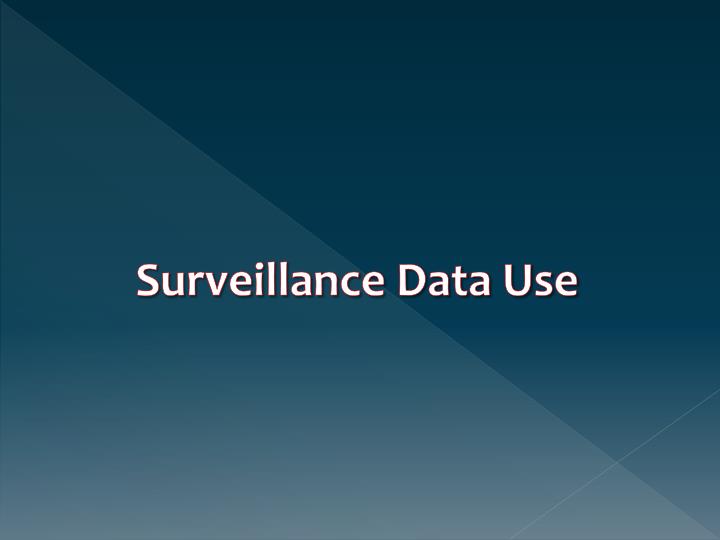The image appears to be a presentation slide with a rectangular shape, divided diagonally from the top left to the bottom right into two contrasting triangles. The upper right triangle is filled with a darker shade of midnight blue, while the lower left triangle features a lighter shade of the same hue, creating a striking visual split. In the very center of the slide, bold white text reads "Surveillance Data Use," making it easy to read. Additionally, there's a thin white line that cuts diagonally across the bottom right corner, further complementing the design. The overall background seems to have a subtle gradient effect from top to bottom, enhancing the visual appeal of the slide.